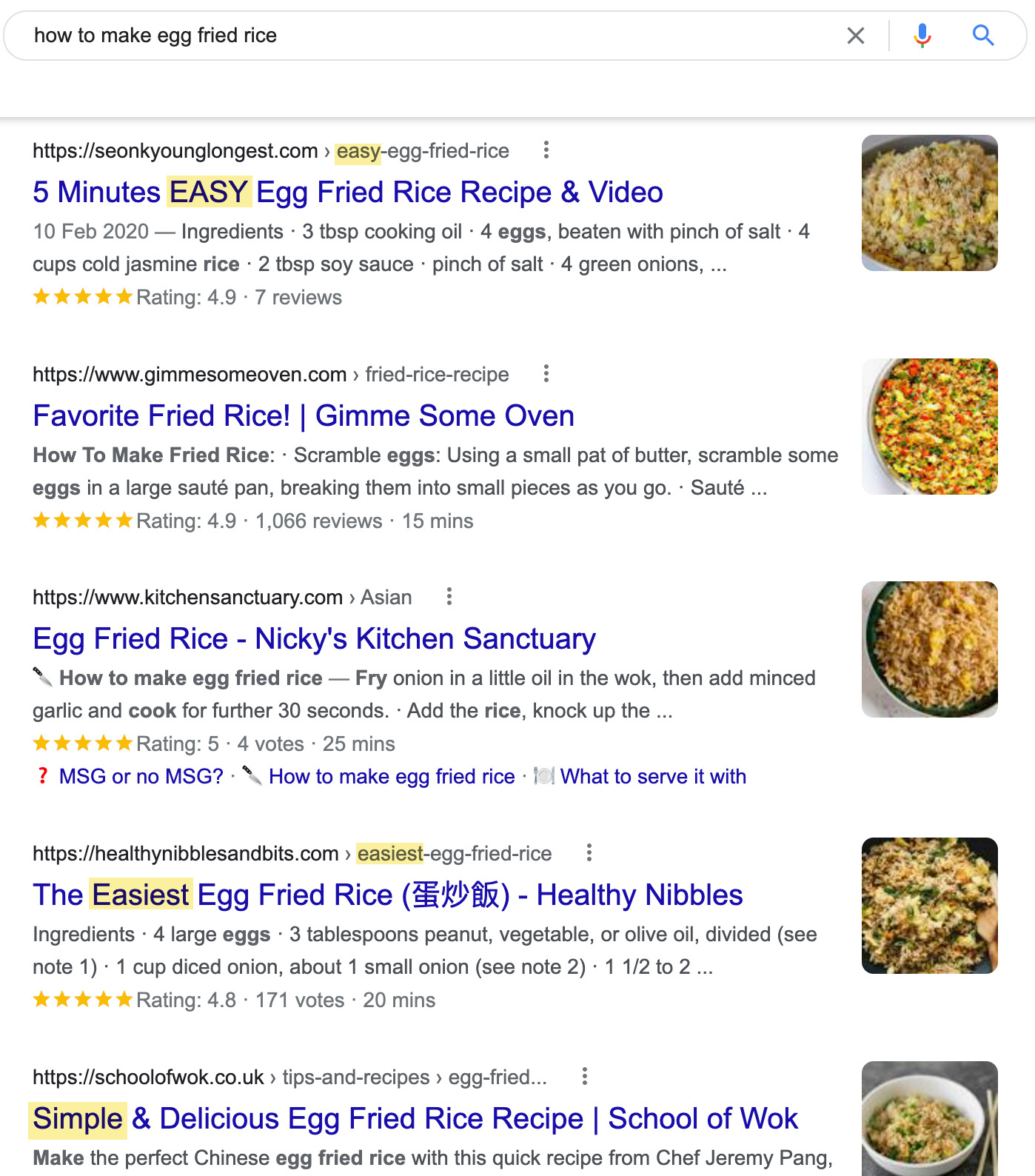**Detailed Caption:**

This image is a screen capture in portrait mode, displaying a web search for "how to make egg fried rice." The screen capture is tall and narrow, featuring a white background. Prominently at the top of the page is the search bar, with five search results listed below it. The text for clickable links is in blue, while descriptions are rendered in black.

The layout aligns all text to the left side of the page. To the right of each search result text block is a small square thumbnail image of the egg fried rice dish. These thumbnails showcase primarily tan and golden rice, accented with the vibrant colors of various vegetables.

The five available links presented are:

1. **5 Minutes Easy Egg Fried Rice Recipe and Video**
2. **Favorite Fried Rice, Gimme Some Oven**
3. **Egg Fried Rice, Nikki's Kitchen Sanctuary**
4. **The Easiest Egg Fried Rice, Healthy Nibbles**
5. **Simple and Delicious Egg Fried Rice Recipe, School of Wok**

Several keywords in these search results are highlighted in yellow: the word "easy" appears twice, "easiest" appears twice, and "simple" appears once. Additionally, yellow accents highlight the star ratings for each search result, contributing to the visual emphasis of the page.